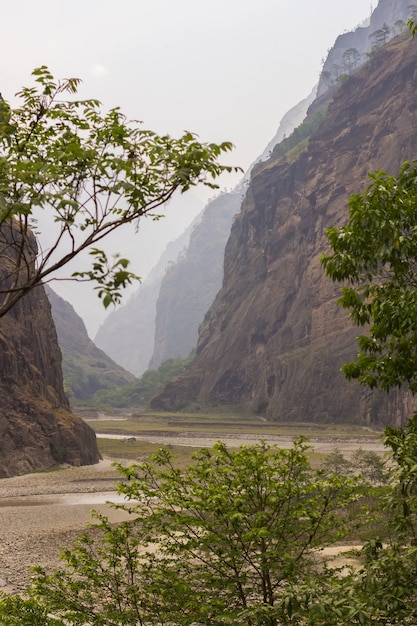This rectangular outdoor photograph, likely taken during a rainy day, captures a serene mountain pass with a winding, shallow brown river meandering through a flat riverbed. The sky is a solid light blue-gray, indicative of a foggy or overcast day. Tall, rocky cliffs dominate the right side of the image, climbing steeply out of frame and adorned with patches of greenery. Flanking the river are deciduous trees and bushes, with one particularly noticeable bush in the foreground. The trees' green foliage contrasts with the rugged cliffs, creating a tranquil and humid atmosphere. Although the exact location is unclear, it evokes landscapes seen in regions such as Africa, Utah, or parts of Asia.